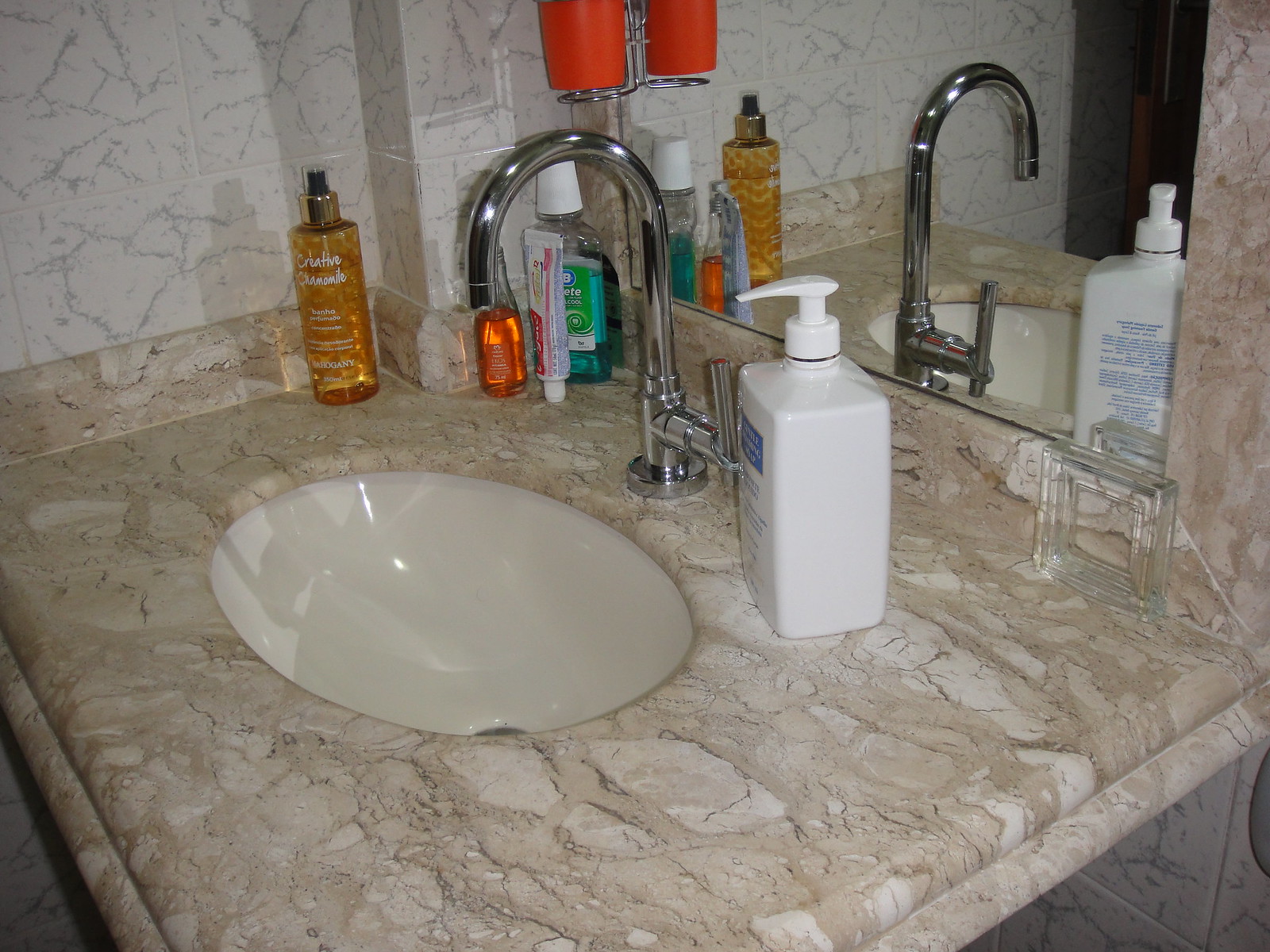This indoor close-up photograph captures the corner of a kitchen countertop, viewed from an angled perspective. Dominating the foreground is a white, under-mount porcelain sink embedded in a luxurious white marble countertop, enhanced with subtle streaks of gray and brown. A sleek chrome faucet, designed as a single stem with an elegant upside-down J-shaped curve, stands prominently behind the sink.

Adding to the scene, a tall rectangular bottle of hand lotion with a side-aligned label is positioned directly in front of the faucet. In the corner background, a tube of toothpaste balances upright on its cap, flanked by a bottle of mouthwash and what appears to be an aftershave bottle. Slightly left of center, another bottle – possibly containing hair gel – stands guard.

The right side of the image features a mirror that partially intrudes into the foreground, reflecting the lighter marble-tiled wall. This wall subtly blends with the countertop, maintaining a cohesive design aesthetic. Lastly, peeking from the upper edge left of center, an orange object—potentially the bottom of a cup—adds a pop of color and a touch of mystery to the composition. The image is devoid of any visible text or print, focusing purely on the arrangement and textures within the scene.